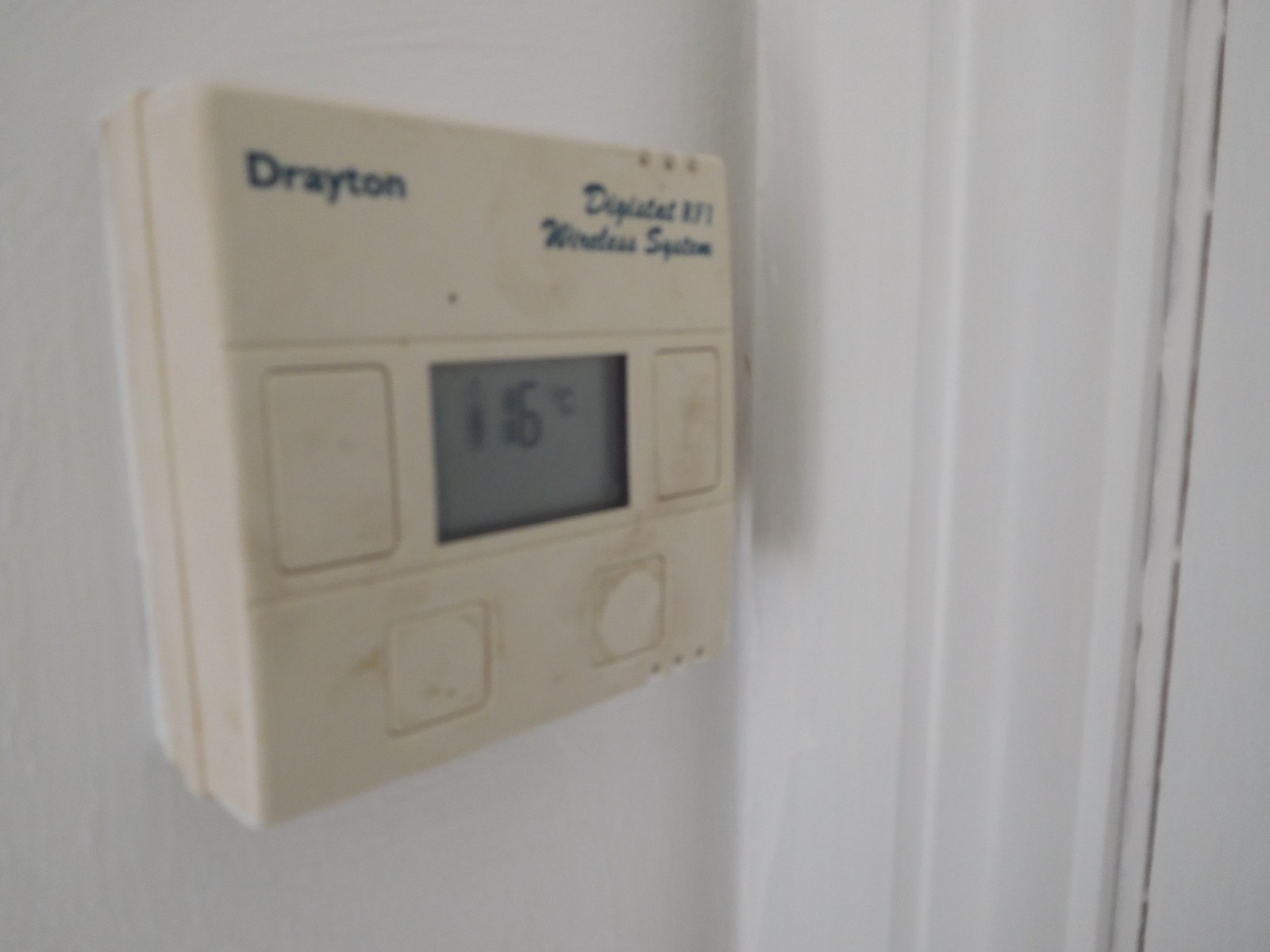The image showcases an old, off-white thermostat mounted on a white wall. The thermostat appears dirty, with visible stains indicating its age and usage over time. The central display window shows an improbable reading of 116°C. The layout includes two large buttons on either side of the display and two smaller buttons positioned below it. The upper left corner is branded with the name "Drayton," while the upper right corner bears the label "Wonder System." Above this label, there are some indistinct and worn-out numbers. Overall, the thermostat's design and condition suggest it is an outdated model.